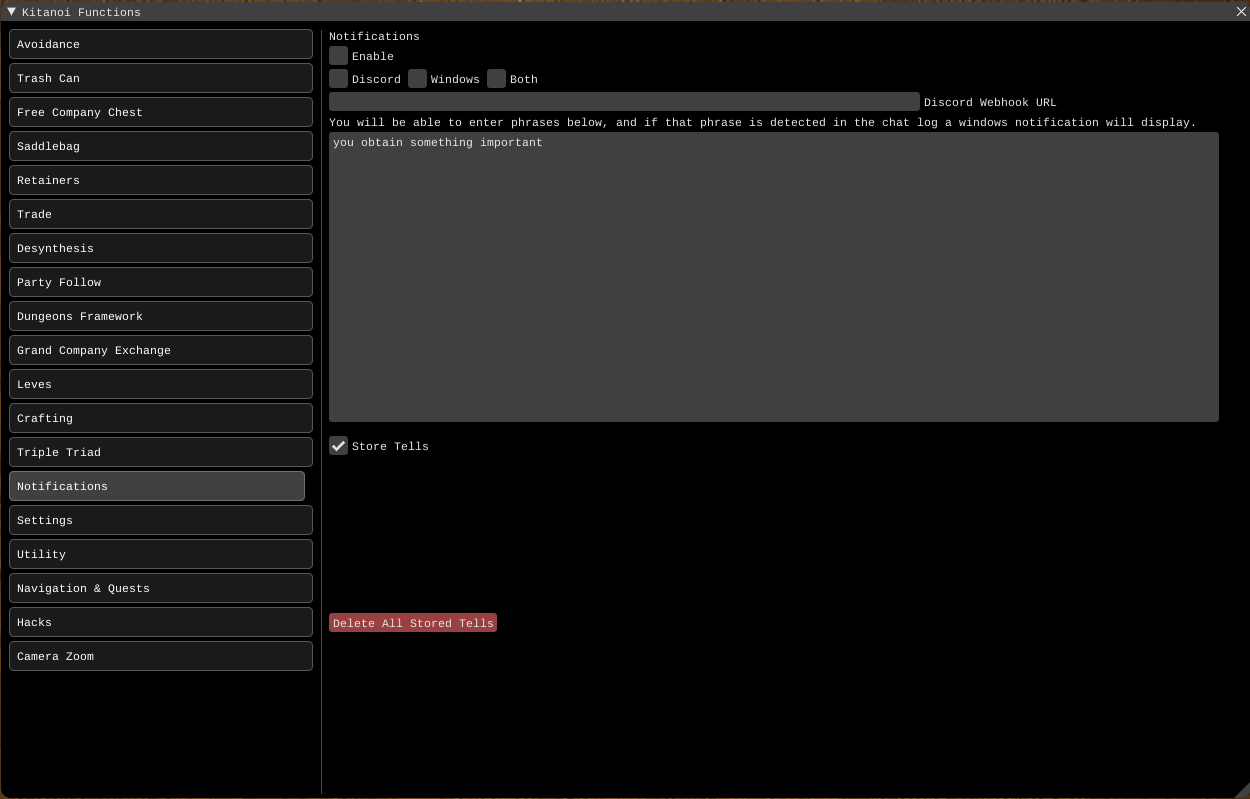This screenshot displays a specific application or plugin that appears to be integrated with Discord and/or Windows, named "Kitanoi Functions". The interface exhibits an extensive list of functionalities on the left-hand side, including:

- Avoidance
- Trashcan
- Free Company Chest
- Saddlebag
- Retainers
- Trade
- Desynthesis
- Party Follow
- Dungeons Framework
- Grand Company Exchange
- Levees
- Crafting
- Triple Triad
- Notifications (which is currently selected)
- Settings
- Utility
- Navigation
- Quests
- Packs
- Camera
- Zoom

The "Notifications" section is highlighted, revealing several options. There is a button to enable notifications, as well as a button to select either Discord, Windows, or both platforms for these notifications. Additionally, there is a field to input a Discord webhook URL. Beneath this, there is a section where one can enter specific phrases. When these phrases are detected in the chat log, a Windows notification will be triggered. An example entry, "you obtained something important," is shown and checked off. At the bottom of this section, there is an option to store incoming messages (referred to as "Store Tells"), as well as a button to delete all stored messages.